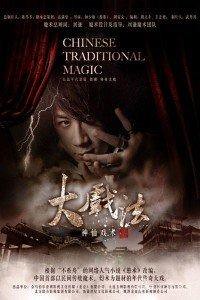A promotional poster for a magic show titled "Chinese Traditional Magic" features an eerie and dark theme. The central figure, a man with longish brown hair styled in an emo fashion, gazes sinisterly at the viewer while extending his fingers, adorned with rings, towards the camera. He is partially obscured by dark burgundy curtains that frame his face. A faint lightning bolt can be seen streaking past his head, adding a mystical element. Surrounding the man are large, yellow Chinese symbols that stand out prominently amidst the dark background. Below him is a blurred depiction of a traditional Chinese city enveloped in smoke or mist, adding to the mysterious atmosphere. The bottom portion of the poster, lighter in color, contains additional rows of language characters, although they are largely illegible due to size and reproduction constraints.